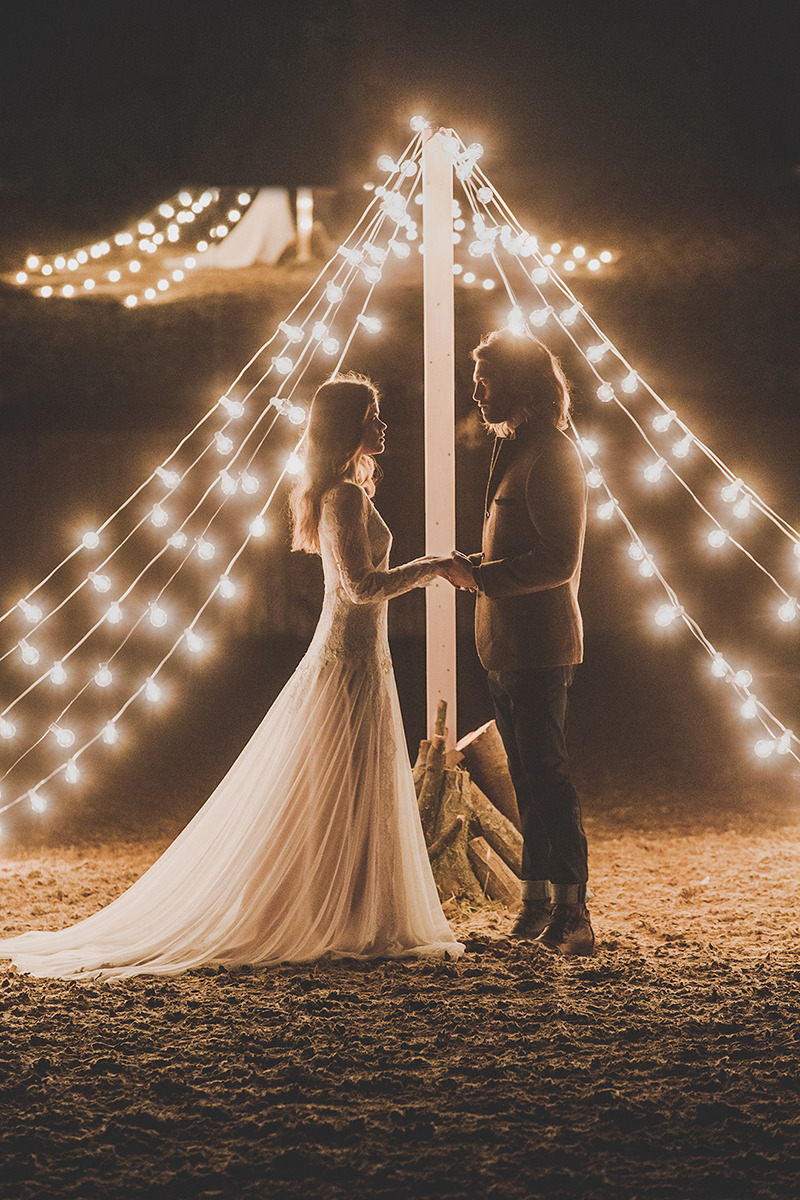This nighttime outdoor photograph captures a newlywed couple standing in front of a softly illuminated tent in a sandy or dirt-filled area. The bride, positioned on the left, is wearing a stunning white wedding gown with long lace sleeves and a delicate, flowy train that trails behind her in the sand. Her long brown hair cascades down to her mid-back, free of any veil or headpiece. The groom, standing on the right, is dressed in a brown suit jacket paired with darker tight-fitting pants and ankle boots. He has shoulder-length brown hair and is gazing intently at his bride while holding her hands. Behind them, a small white column adorned with lights supports the lit canopy, adding a romantic glow to the scene. The background reveals a tent adorned with string lights, enhancing the celebratory atmosphere of this special moment.